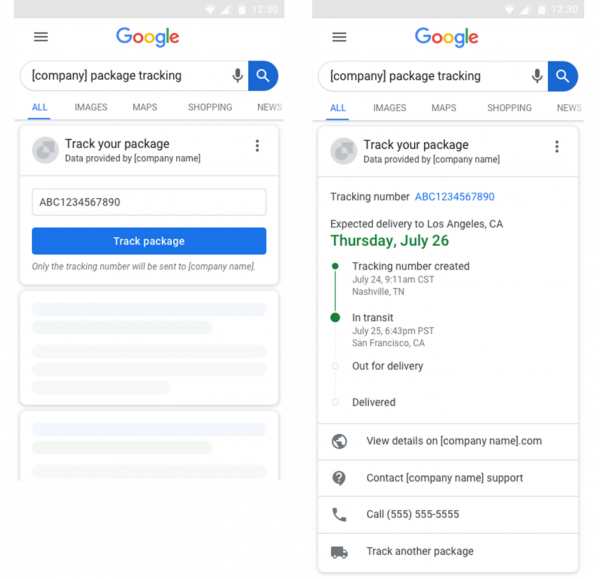This image consists of two screenshots of mobile phones placed side-by-side, each displaying a package tracking interface. 

The first screenshot, located on the left, features a gray status bar at the top showing the time as 12:30 and the battery life. Below this, a hamburger menu icon is located on the top left corner. In the center, it prominently displays the Google logo above a search bar. Underneath, it reads "company package tracking" inside the search bar. Further down, a navigation menu contains options such as "All," "Images," "Map," "Shopping," and "News." The main part of the screen provides package tracking information: a prompt to "Enter Tracking Number," displaying an example tracking number "ABC1234567890." A blue "Track Package" button is visible below this, but the remainder of the screenshot doesn't show any additional content.

The second screenshot on the right mirrors the format of the first, with identical elements along the top, including the status bar, hamburger menu, Google logo, and search options. The search bar also indicates "company package tracking," and the same tracking number "ABC1234567890" appears. Below this, the package updates are displayed. It indicates that the package is expected to be delivered to Los Angeles, California, on Thursday, July 26, with the date highlighted in green. The tracking information includes the following statuses: "Tracking Number Created," "In Transit" (highlighted in green), "Out for Delivery," "Delivered," and a prompt to "Track Another Package." Further options to "View Details on Company Name.com" and "Contact Company Name Support" provide a phone number formatted as "555-555-5555." The interactive elements and detailed tracking statuses distinguish this screen from the first, providing comprehensive package tracking details.